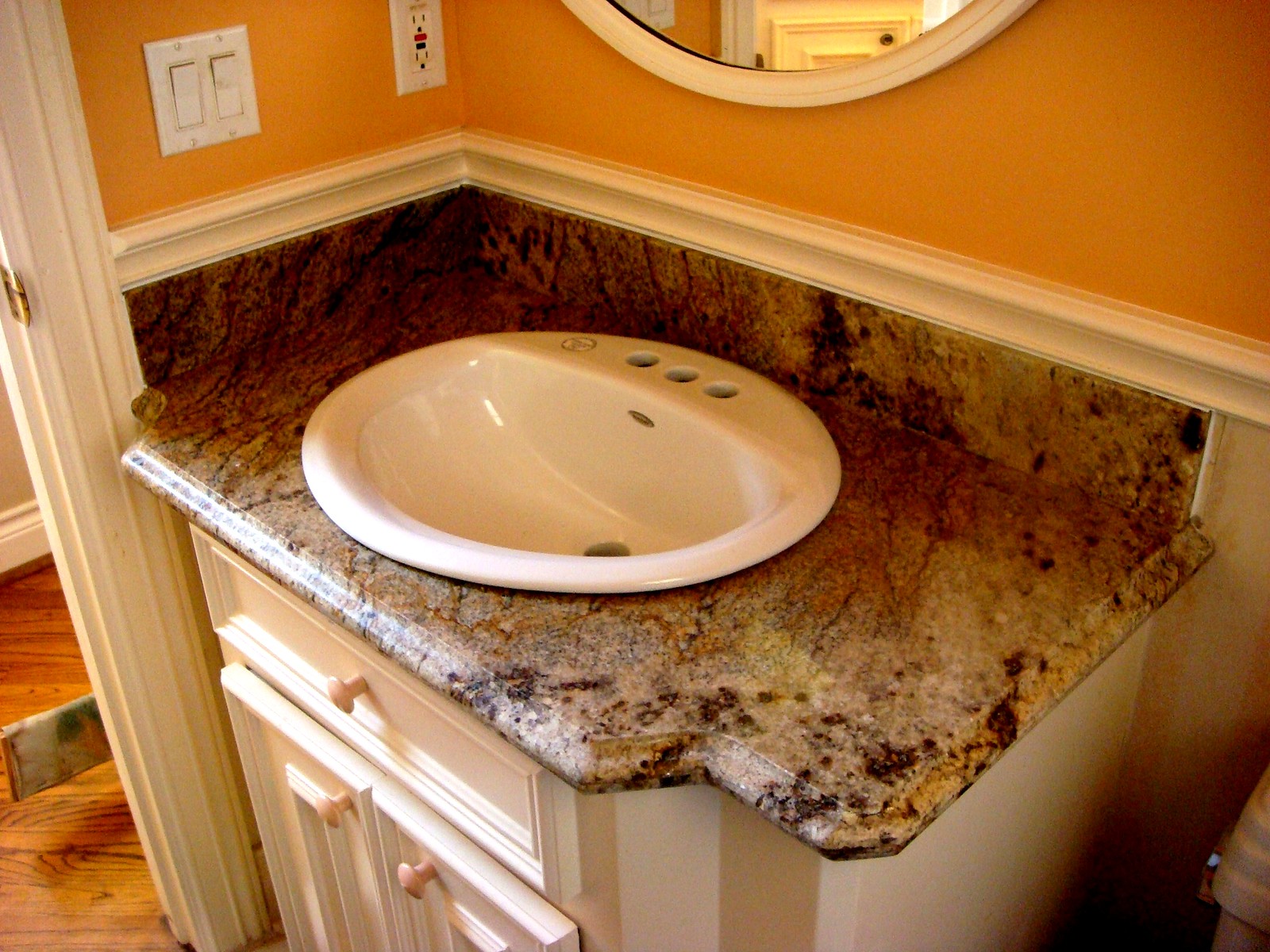This image captures a bathroom in the midst of its setup, focusing on the sink and counter area. The marble countertop, a pristine white with subtle veining, is yet to be fully equipped, as evidenced by the absence of both the faucet and handles on the sink. The base of the counter is designed with a sleek, minimalist aesthetic, featuring a single drawer and two cabinet doors, all painted in white. The wall behind showcases a bold orange hue, accentuated by a white trim running vertically down the center.

Partially visible is the bottom section of a circular mirror, bordered in white, that promises to add a touch of elegance upon completion. Nearby, a dual-panel white light switch and an adjacent electrical outlet with two open slots are installed, ready for use. To the far left of the image, a doorway framed by a wooden floor leads out to a hallway, where some construction materials hint at ongoing renovation work. On the extreme right, the very edge of a toilet and its handle are just visible, indicating the restroom's progress towards finalization.